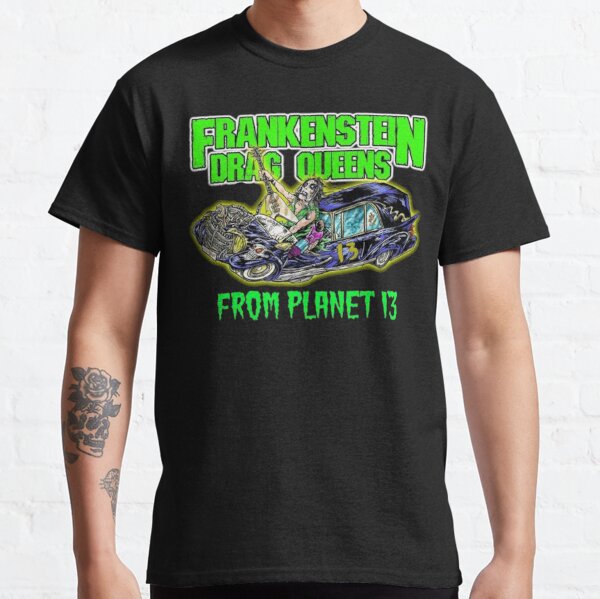This square photograph captures a person standing in front of a white painted brick wall, showcasing a striking black t-shirt. The image is carefully cropped to include only the person's neck, arms, and upper torso, thereby focusing the viewer's attention solely on the t-shirt. The shirt itself is a short-sleeve, crew neck design, emblazoned with neon green, all-caps text at the top stating "FRANKENSTEIN DRAG QUEENS," outlined in white for emphasis. Below the text, there's an eye-catching graphic of a zombie-like figure wielding a guitar inside a hearse-style car. Further enhancing the design, the words "FROM PLANET 13" appear in neon green beneath the image, featuring a drip effect that adds to the eerie aesthetic. The person’s right forearm is visible, displaying a black tattoo of a skull adorned with flowers, while another indistinct tattoo is partially visible on the underside of the same arm. This detailed composition effectively highlights the unique and bold design of the t-shirt against the stark, white brick wall backdrop.